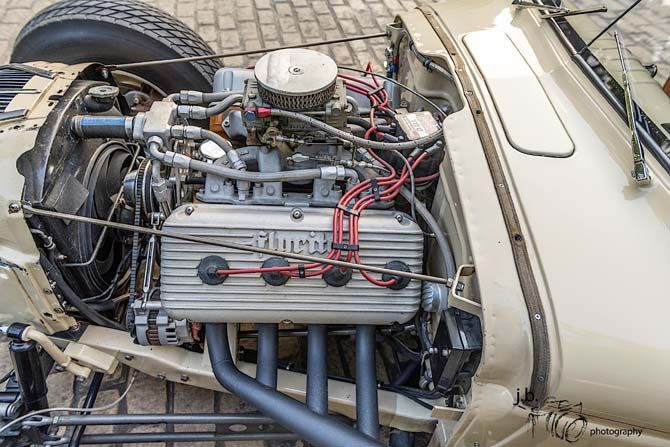This is a detailed color photograph of the exposed engine compartment of an old-fashioned car, likely a hot rod from the 1940s or 1950s. The vehicle, which is brown, is parked on a cobblestone surface. The hood has been removed, revealing a complex array of components. Prominently visible in the upper right corner are the windshield and its angled wipers, slanted upward and inward toward each other. The engine itself features a big silver cover and a silver air filter on top, alongside various black, gray, and blue pipes and hoses extending in multiple directions. Red and off-yellow wires are intertwined throughout the setup. Notable details include a gray box on the side with four red metal wire-like straws emerging from black circles, and a set of exhaust pipes leading out. The engine bears a partially visible brand or model name: FLYRITE. Additional details captured include a black fan in front of a black radiator, and a visible tire. In the bottom right corner of the image, small gray letters spell out "J. B. Photography."